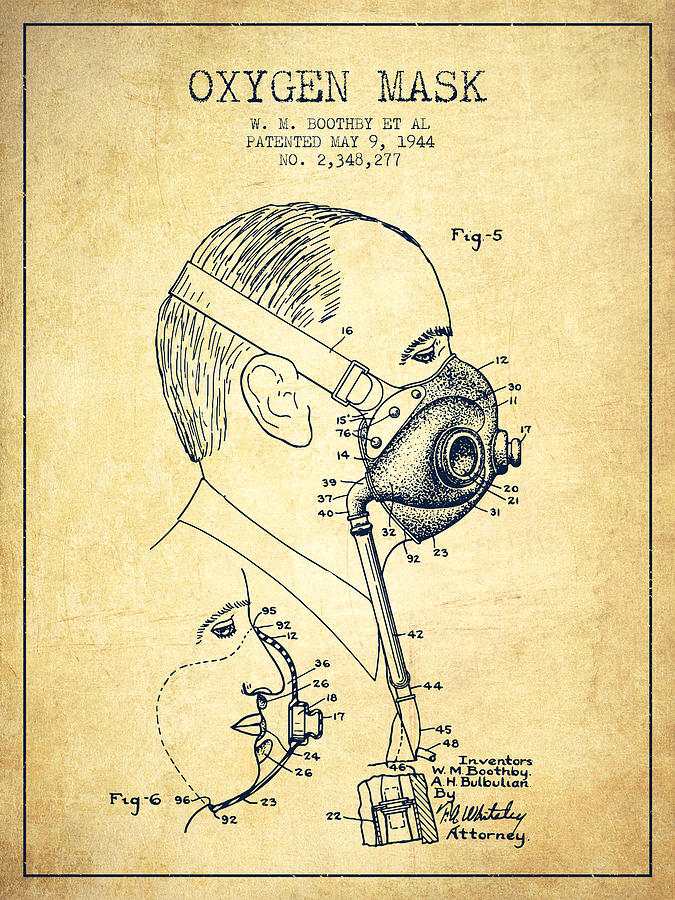This is an aged and weathered illustration from a medical text or patent application, rendered on tan, almost scroll-like paper with a thin black outline bordering the entire image. At the top, in a typewriter font, it reads "OXYGEN MASK" followed by "W. M. Boothby, et al. Patented May 9, 1944, Number 2,348,277." Below this header, the main illustration labeled "Figure 5" depicts a man in profile, facing right, wearing an oxygen mask. The mask, drawn in black ink with a white headband, covers his nose and mouth, with various parts labeled by numbered lines that seem to correspond to a legend not visible in the image. Surrounding the man’s profile, additional detailed sketches of the mask show an X-ray-like view, indicating the internal workings and placement of each component. The signatures of the inventors, "W.M. Boothby" and "A.H. Bullion," as well as the name of an attorney, "Phil Whitley," are inscribed at the bottom in cursive.